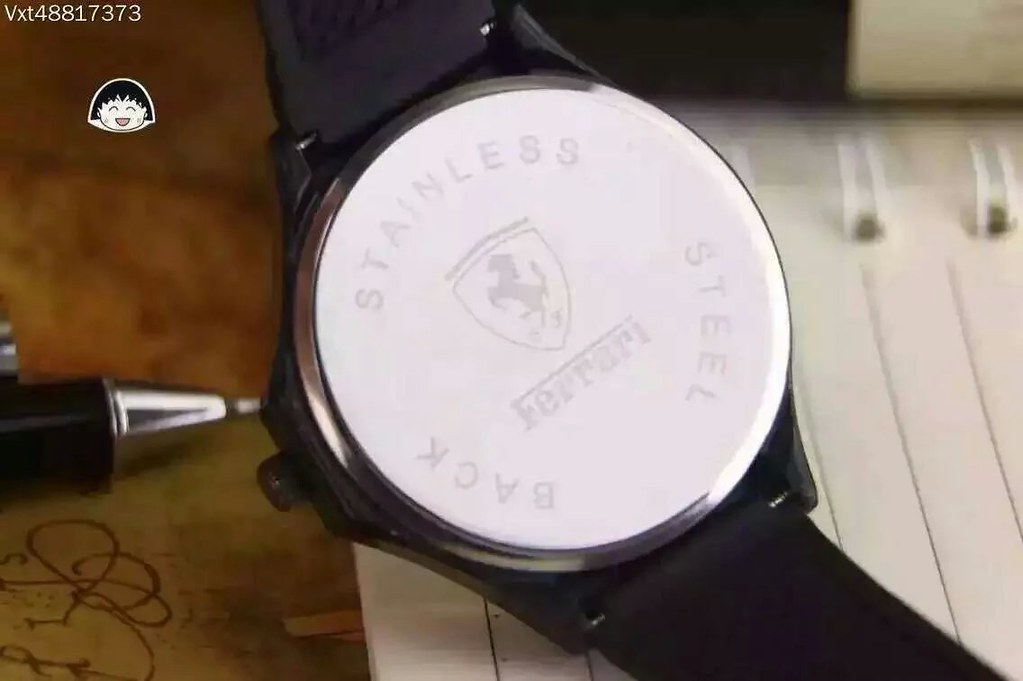- - - - - - - - - - - - - - - - - - - - - - - - - - - - - - - - - - - - - - - - - - - - - - - - - - - - - - - - - - - - - - - - - - - - - - - - - - - - - - - - - - - - - - - - - - - - - - - - - - - - - - - - - - - - - - - - - - - - - - - - - - - - - - - - - - - - - - - - - - - - - - - - - - - - - - - - - - - - - - - - - - - - - - - - - - - - - - - - - - - - - - - - - - - - - - - - - - - - - - - - - - - - - - - - - - - - - - - - - - - - - - - - - - - - - - - - - - - - - - - - - - - - - - - - - - - - - - - - - - - - - - - - - - - - - - - - - - - - - - - - - - - - - - - - - - - - - - - - - - - - - - - - - - - - - - - - - - - - - - - - - - - - - - - - - - - - - - - - - - - - - - - - - - - - - - - - - - - - - - - - - - - - - - - - - - - - - - - - - - - - - - - - - - - - - - - - - - - - - - - - - - - - - - - - - - - - - - - - - - - - - - - - - - - - - - - - - - - - - - - - - - - - - - - - - - - - - - - - - - - - - - - - - - - - - - - - - - - - - - - - - - - - - - - - - - - - - - - - - - - - - - - - - - - - - - - - - - - - - - - - - - - - - - - - - - - - - - - - - - - - - - - - - - - - - - - - - - - - - - - - - - - - - - - - - - - - - - - - - - - - - - - - - - - - - - - - - - - - - - - - - - - - - - - - - - - - - - - - - - - - - - - - - - - - - - - - - - - - - - - - - - - - - - - - - - - - - - - - - - - - - - - - - - - - - - - - - - - - - - - - - - - - - - - - - - - - - - - - - - - - - - - - - - - - - - - - - - - - - - - - - - - - - - - - - - - - - - - - - - - - - - - - - - - - - - - - - - - - - - - - - - - - - - - - - - - - - - - - - - - - - - - - - - - - - - - - - - - - - - - - - - - - - - - - - - - - - - - - - - - - - - - - - - - - - - - - - - - - - - - - - - - - - - - - - - - - - - - - - - - - - - - - - - - - - - - - - - - - - - - - - - - - - - - - - - - - - - - - - - - - - - - - - - - - - - - - - - - - - - - - - - - - - - - - - - - - - - - - - - - - - - - - - - - - - - - - - - - - - - - - - - - - - - - - - - - - - - - - - - - - - - - - - - - - - - - - - - - - - - - - - - - - - - - - - - - - - - - - - - - - - - - - - - - - - - - - - - - - - - - - - - - - - - - - - - - - - - - - - - - - - - - - - - - - - - - - - - - - - - - - - - - - - - - - - - - - - - - - - - - - - - - - - - - - - - - - - - - - - - - - - - - - - - - - - - - - - - - - - - - - - - - - - - - - - - - - - - - - - - - - - - - - - - - - - - - - - - - - - - - - - - - - - - - - - - - - - - - - - - - - - - - - - - - - - - - - - - - - - - - - - - - - - - - - - - - - - - - - - - - - - - - - - - - - - - - - - - - - - - - - - - - - - - - - - - - - - - - - - - - - - - - - - - - - - - - - - - - - - - - - - - - - - - - - - - - - - - - - - - - - - - - - - - - - - - - - - - - - - - - - - - - - - - - - - - - - - - - - - - - - - - - - - - - - - - - - - - - - - - - - - - - - - - - - - - - - - - - - - - - - - - - - - - - - - - - - - - - - - - - - - - - - - - - - - - - - - - - - - - - - - - - - - - - - - - - - - - - - - - - - - - - - - - - - - - - - - - - - - - - - - - - - - - - - - - - - - - - - - - - - - - - - - - - - - - - - - - - - - - - - - - - - - - - - - - - - - - - - - - - - - - - - - - - - - - - - - - - - - - - - - - - - - - - - - - - - - - - - - - - - - - - - - - - - - - - - - - - - - - - - - - - - - - - - - - - - - - - - - - - - - - - - - - - - - - - - - - - - - - - - - - - - - - - - - - - - - - - - - - - - - - - - - - - - - - - - - - - - - - - - - - - - - - - - - - - - - - - - - - - - - - - - - - - - - - - - - - - - - - - - - - - - - - - - - - - - - - - - - - - - - - - - - - - - - - - - - - - - - - - - - - - - - - - - - - - - - - - - - - - - - - - - - - - - - - - - - - - - - - - - - - - - - - - - - - - - - - - - - - - - - - - - - - - - - - - - - - - - - - - - - - - - - - - - - - - - - - - - - - - - - - - - - - - - - - - - - - - - - - - - - - - - - - - - - - - - - - - - - - - - - - - - - - - - - - - - - - - - - - - - - - - - - - - - - - - - - - - - - - - - - - - - - - - - - - - - - - - - - - - - - - - - - - - - - - - - - - - - - - - - - - - - - - - - - - - - - - - - - - - - - - - - - - - - - - - - - - - - - - - - - - - - - - - - - - - - - - - - - - - - - - - - - - - - - - - - - - - - - - - - - - - - - - - - - - - - - - - - - - - - - - - - - -")

Caption:
The upper portion of the image prominently features the model number "VXT 488117373." Adjacent to this is a small symbol depicting a stylized face with a black bowl cut hairstyle, a white face, a pink mouth, and half-arched eyes. To the bottom left of this symbol, there is a brown area where a pen with a silver tip is placed. Continuing to the left, a stainless steel Ferrari watch is visible, showing the backplate and the iconic Ferrari logo featuring a rearing horse inside a shield. The watch has black leather straps that are slightly flecked around the edges. Below the watch, a brown leather notepad or notebook is placed, topped with rings and showing some scribble marks near where the pen rests. The overall arrangement suggests a desk setup with various personal items.